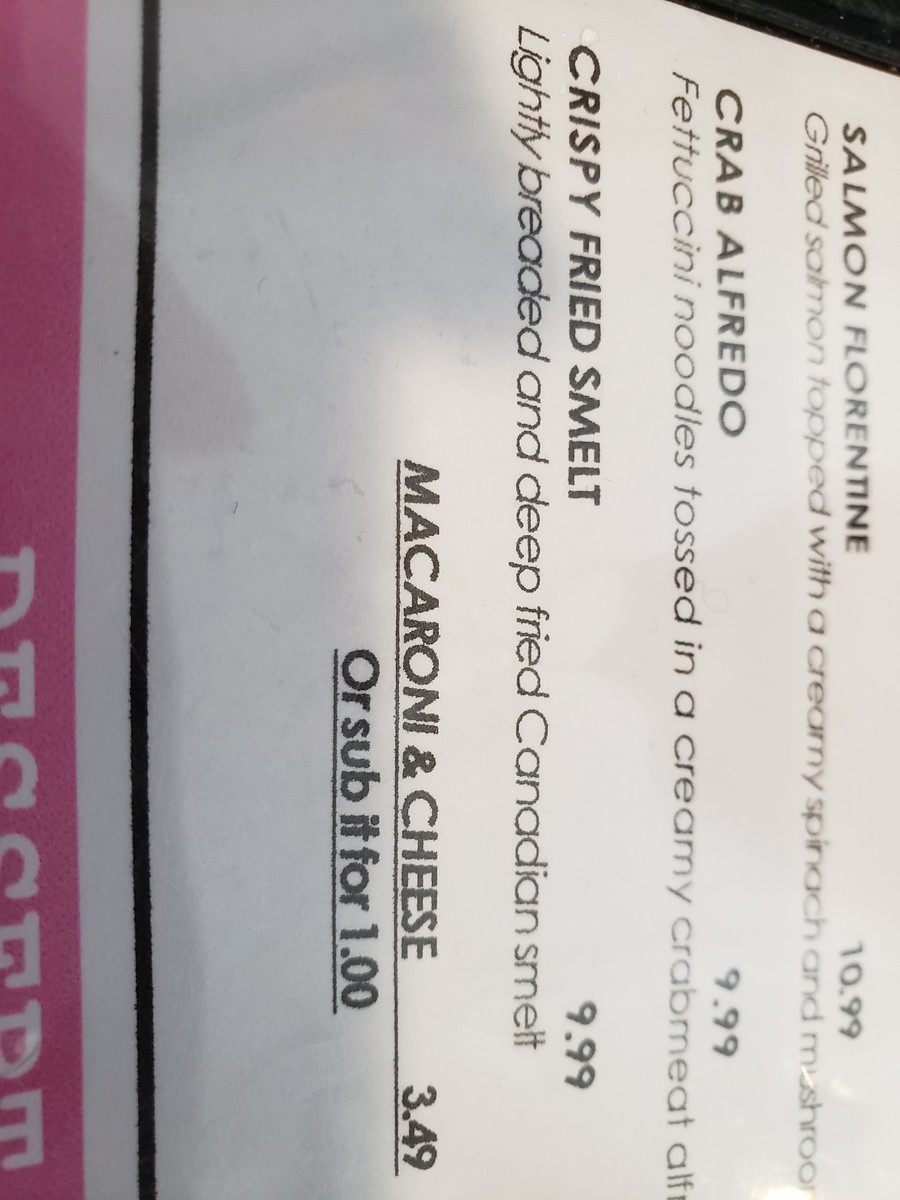This close-up photograph captures a portion of a menu, presented sideways with the text's top aligned to the right and bottom to the left. The menu itself extends beyond the photo's edges in all directions. In the upper right corner, a thin black triangle is visible, likely the edge of the menu or the table beneath it. The menu is printed on white paper and shaded with gray on the left half. Along the far left edge, a strip of pink runs vertically, marked with the white text "DESSERT," partially visible with the lower portion cut off by the photo's edge.

Above the pink strip is a thin black line, separating it from the main text area, which lists dishes in bold, all-caps format. The listed items include "SALMON FLORENTINE," "CRAB ALFREDO," and "CRISPY FRIED SMELT," each followed by a non-bolded description and prices positioned at the photo's bottom due to the rotated orientation. The prices are $10.99, $9.99, and $9.99 respectively. In the lower left of the menu, there is a bold and underlined section reading "MACARONI AND CHEESE," priced at $3.49, with an option to substitute it for $1.